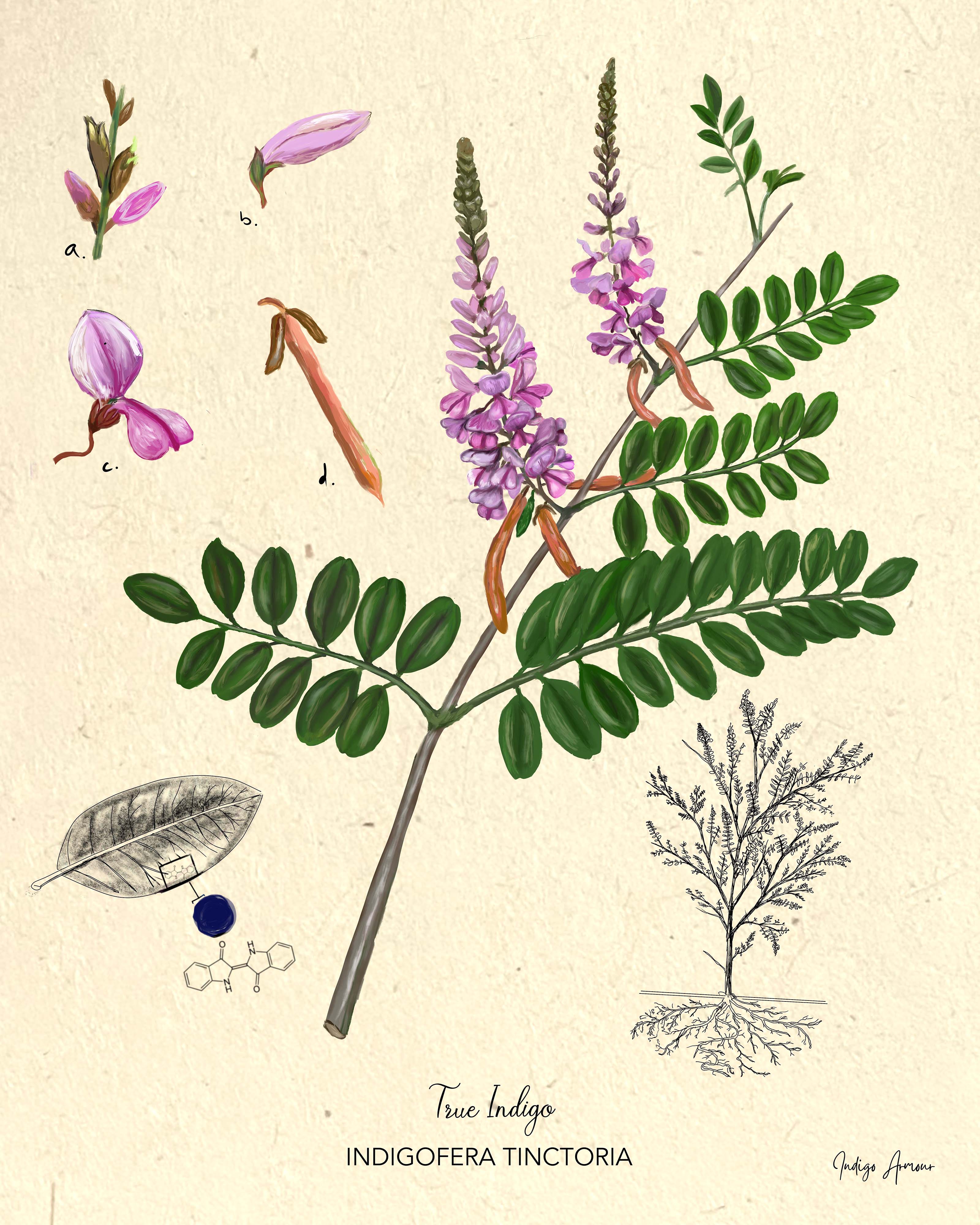The image appears to be a very detailed and educational poster or a page from a botanical book. Dominating the poster is a central illustration of a plant labeled with the letters A, B, C, and D in the top left corner. This plant features a full stem, adorned with leaves and clusters of pinkish flowers. The detailed depiction of the stem shows it branching out with multiple leaves on both sides leading up to the flowers. 

On the bottom left of the poster, there is a black and white drawing of a single leaf, accompanied by what seems to be a cellular diagram within a blue circle. To the right of this section, there’s another illustration showing a black and white rendering of the entire plant or tree.

At the very bottom of the poster, the text reads "True Indigo" and underneath that, "Indigofera tinctoria," identifying the scientific name of the plant. Additionally, there is a signature in the bottom right corner, though it is not legible. The background of the poster has a pinkish blush hue, with an informative and scientific layout, possibly making it suitable for educational purposes, such as a children's science project.